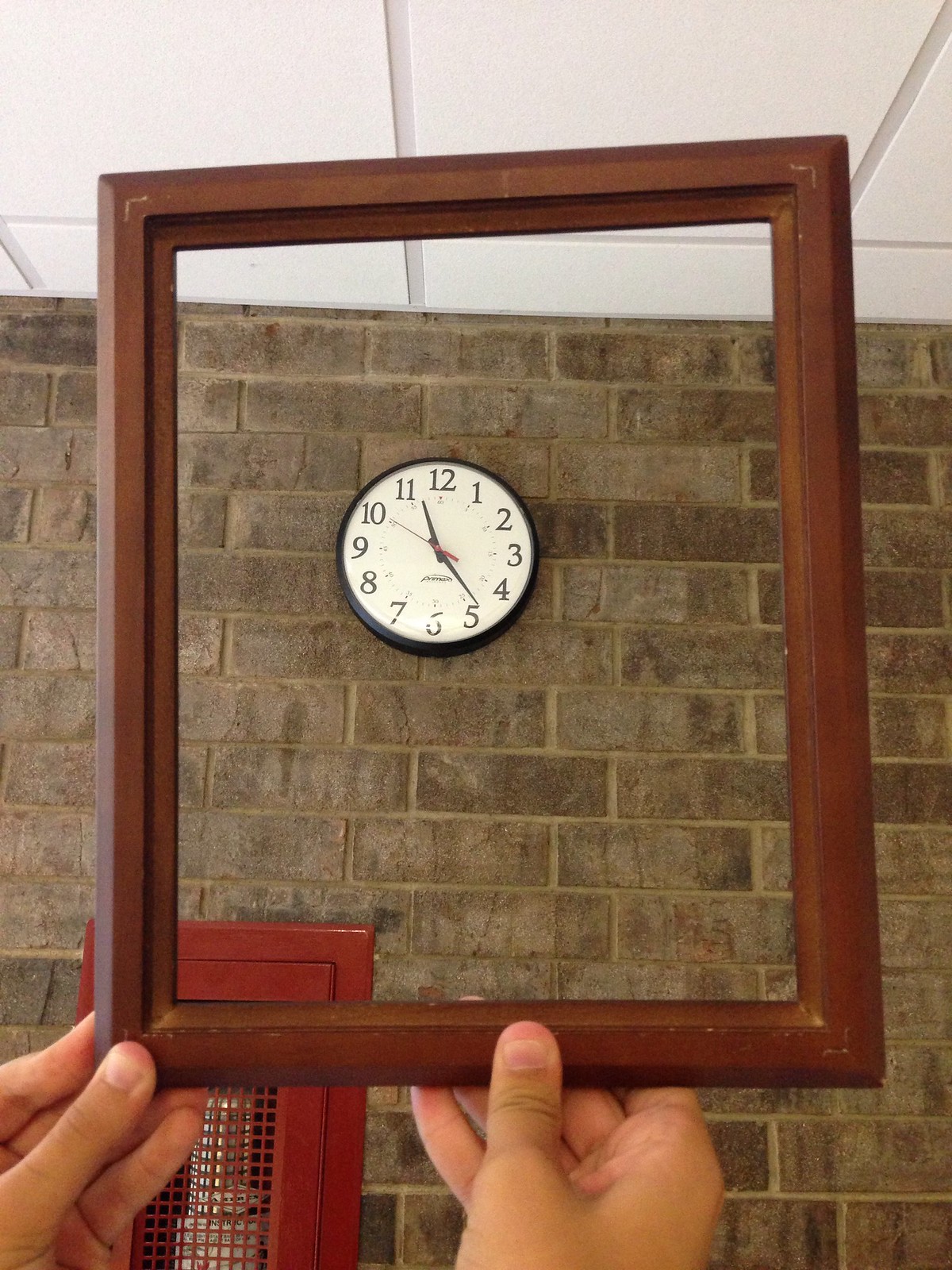This color photograph showcases an empty brown picture frame held up by a person's hands in the foreground, framing a round wall clock behind it. The clock, situated on a brick wall composed of varying shades of gray bricks, features a black frame, a white face, large black numbers, and black hands indicating approximately 11:24, with the second hand at 10. The brick wall backdrop creates a stark contrast with the clock, enhancing its visibility. The ceiling is white with drop ceiling tiles. Additionally, a red-framed, caged fire extinguisher is visible at the bottom left corner of the image, integrated into the wall. The photograph is taller than it is wide, not featuring any signs, text, animals, plants, flowers, or trees.